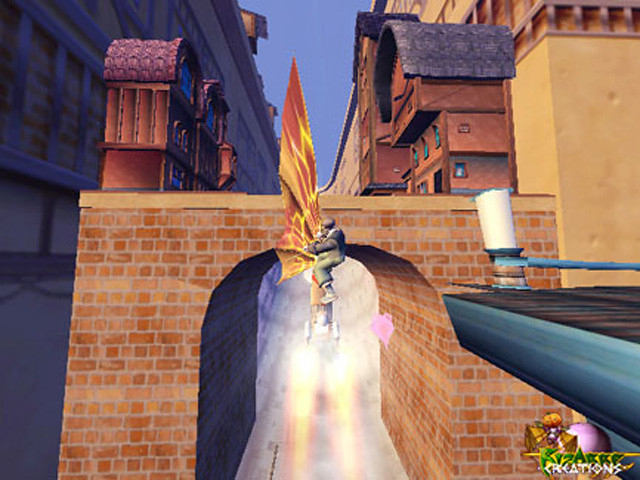The image depicts a computer-generated scene from a video game, focusing on a person riding a rocket-powered surfboard. The surfboard, which has two rockets attached to its underside emitting fiery jets of red and yellow, also features a single, triangular, butterfly-like wing on top, colored in shades of red, yellow, and light tan. The rider is dressed in a brown coat and green pants and is gripping the wing while soaring towards a stone archway between two brown structures with rounded roofs. The structure on the right has a grayish roof, while the one on the left has a reddish roof. There is a waterway flowing beneath the arch, disappearing into a tunnel. On the bottom right of the image, part of another roof with blue trim is visible, while on the upper right, a light brown building stands adjacent to the brick structure. To the left, a darker bluish-gray building can also be seen.